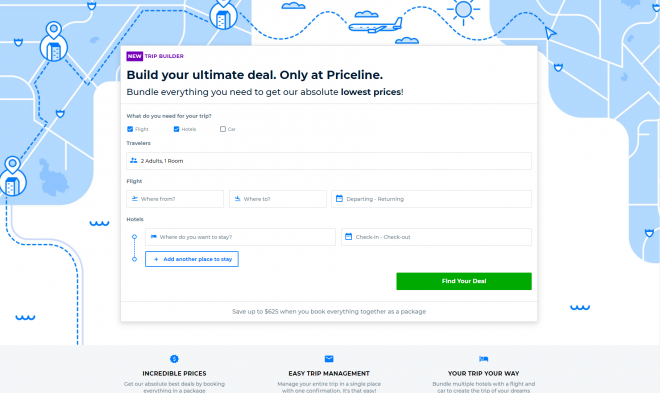The image showcases a web page displayed on a computer monitor, featuring Priceline's Trip Builder tool. The background resembles a simplistic, cartoon-like map. In the center of the screen, a prominent pop-up appears with the header "New Trip Builder," inviting users to "Build your ultimate deal only at Priceline." The pop-up encourages bundling all necessary travel components to secure the absolute lowest prices. 

The interface includes a series of checkboxes under the prompt, "What do you need for your trip?" with options like "Flight" and "Hotel" marked as selected. The traveler details specify "Two adults" and "One room, flight." There are input fields for specifying departure and destination locations, as well as departure and return dates. Additional sections allow users to select their hotel preferences with "Check-in" and "Check-out" dates, and an "Add" button to include another accommodation.

At the bottom of the pop-up, a bold green button labeled "Find Your Deal" encourages users to proceed. Supplementing the main content are three highlighted sections at the page's bottom, albeit partially obscured. These sections tout benefits under the headings "Incredible Prices," "Easy Trip Management," and "Your Trip Your Way," accompanied by descriptive text that is not entirely legible.